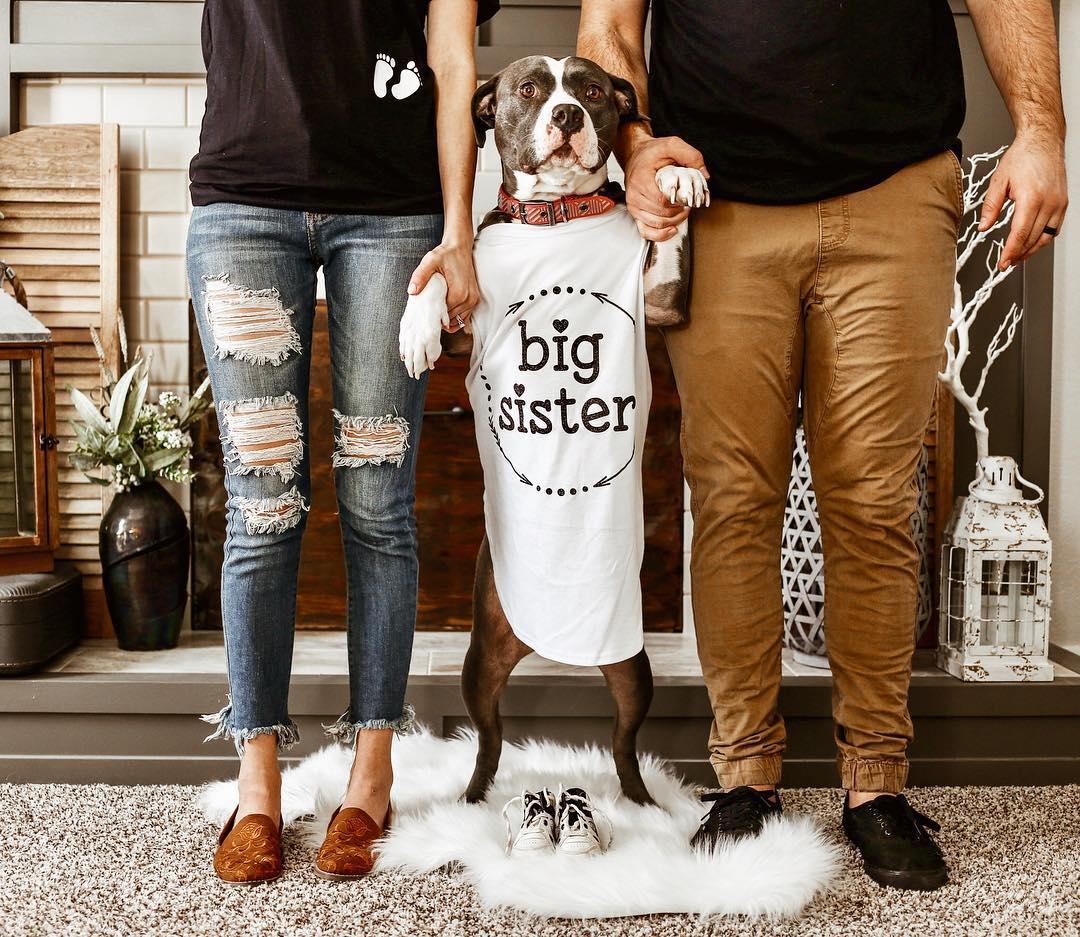A detailed photograph captures a man and a woman holding a female dog between them, standing in front of a hearth with a farmhouse aesthetic. The hearth features a beige brick facade and is decorated with a distressed white lantern and white branches in a vase. From the waist down, both the man and woman are visible, each holding one of the dog's front paws as it stands on its hind legs on a white faux fur throw rug atop a beige and white carpet.

The woman, positioned on the left, is dressed in a black t-shirt with a design of white baby footprints on the bottom left, paired with weathered, distressed jeans and orange slip-ons with no socks. To her left stands a vase filled with white flowers. The man, standing on the right, wears a black shirt, brown cargo pants that gather at the ankles, and black shoes, also without socks.

The dog, with a cute, surprised expression on its face, wears a red collar and a t-shirt emblazoned with the words "Big Sister" in black text. The dog's coat features a mix of colors, with white on its nose and forehead, and a blend of dark brown and almost grayish hues on its face. At the dog's feet, a pair of white baby shoes can be seen, adding to the heartwarming family scene.